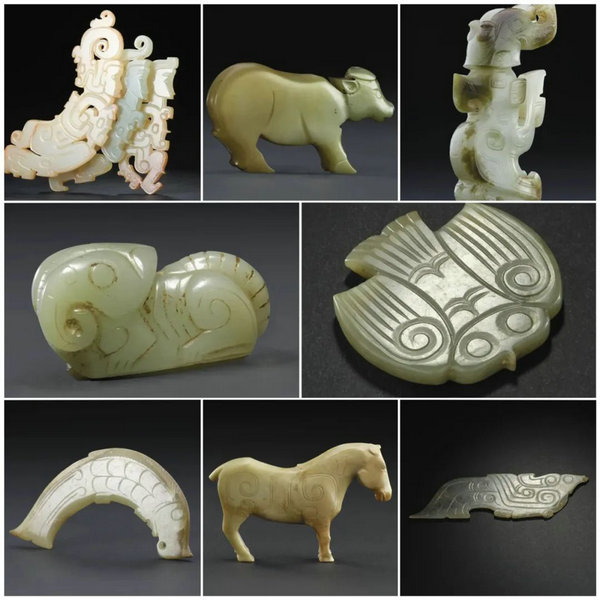This detailed photographic image shows a carefully arranged series of eight small photos featuring various artifacts, likely of Inca, Aztec, or ancient Native American origin. The artifacts, primarily made of jade, are set against a charcoal gray or black background and are separated by thin white lines. The layout includes three square-shaped images at the top, followed by two rectangular ones in the middle, and another three square ones at the bottom. 

In the top left, there are three curved jade pieces—two yellow and one green—that resemble earrings with faces of people. To the right is a small jade figurine of what looks like a pig, and further right, another standing jade piece resembling a fanciful animal with its head turned away. 

On the left of the middle row sits another fanciful jade piece, possibly depicting a creature with an elephant-like trunk and large eye. Adjacent to it is a small jade figure that evocatively resembles a stylized owl, identifiable by its wings, tail, and eyes.

The bottom row features, from left to right, a jade artifact shaped like a fish in an upside-down 'U' form, a jade horse with short legs looking left to right, and a parallelogram-shaped jade piece with intricate swirls and lines, potentially an arm bracelet or piece of jewelry.

The entire arrangement is both visually striking and meticulously detailed, highlighting the intricate craftsmanship of these fascinating ancient artifacts.